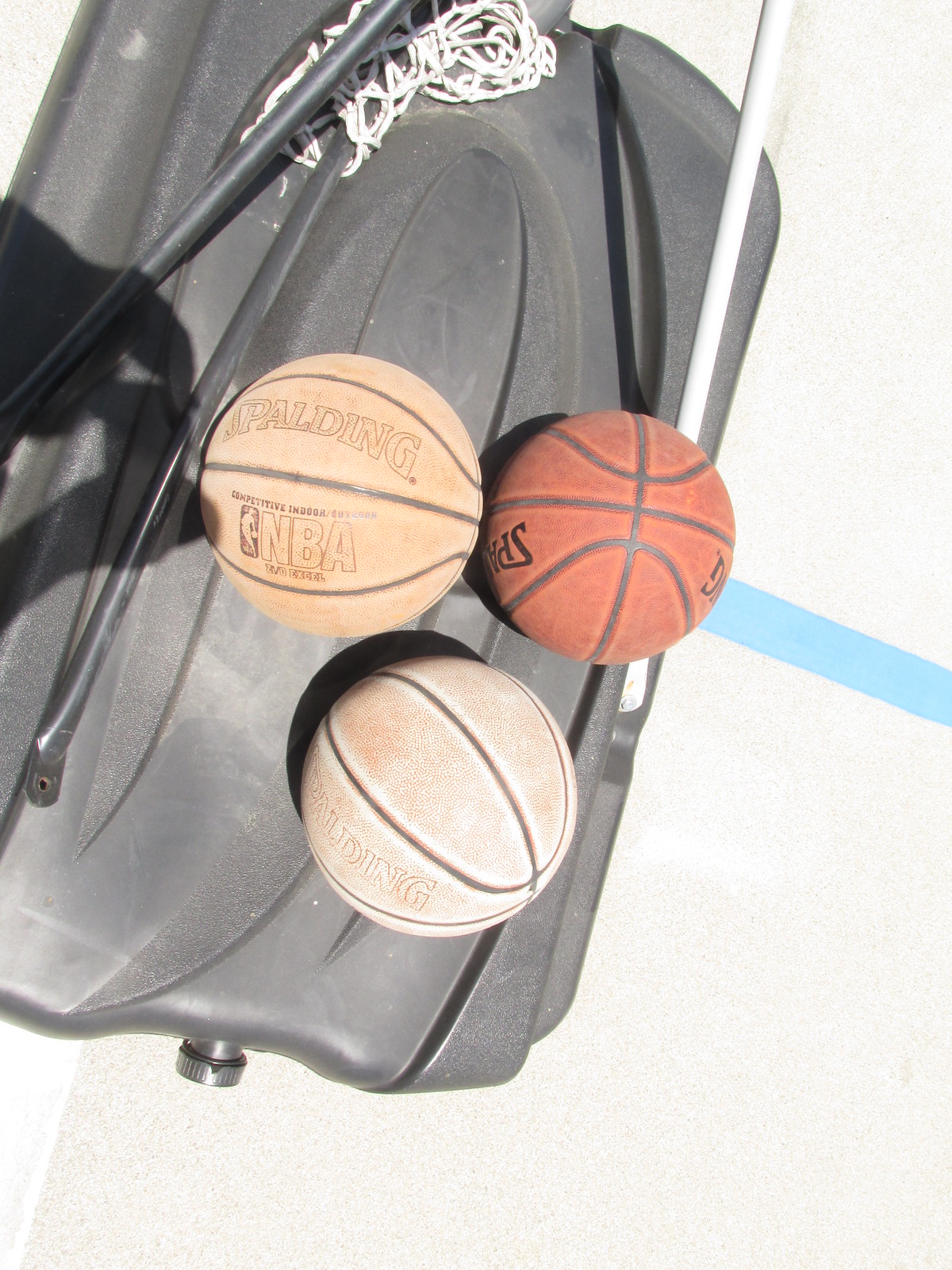This vibrant color photograph captures the bottom section of a portable basketball hoop, specifically its black, slightly worn base, set outdoors in what appears to be a driveway or yard. The net from the hoop lies collapsed on top of the base, indicating that the hoop has not been extended for use. Three basketballs, all Spalding brand, rest on the base. Positioned centrally is a bright orange basketball, appearing almost brand new. To its left is another Spalding ball, duller in color, bearing the words "NBA" and showing significant signs of sun exposure, resulting in a yellowish-brown hue. Below these two is the third basketball, markedly faded and worn, with an off-white color hinting at extensive use and weathering. The image angles to focus on these three basketballs, highlighting the contrast in their conditions against the backdrop of the black, worn base, which also features a visible blue line.